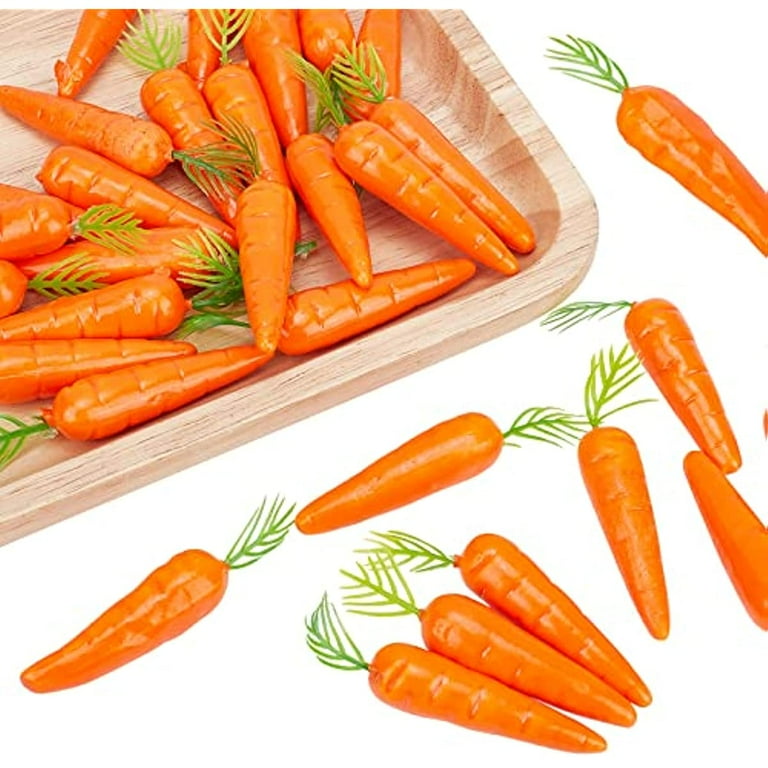This image captures a collection of vibrant baby carrots arranged in a light wood tray and scattered across a white surface. The carrots, each approximately 3-8 inches in length, are uniformly shaped with visible lines running through their shiny orange exterior, likely suggesting they may have been either polished or cooked, enhancing their glossy look. All the carrots feature a small green frond at the top, contributing to a realistic and appealing presentation. The shallow wooden tray, with its natural grain visible and hues of white, tan, and beige, holds the majority of these carrots, adding a rustic charm to the setup. This detailed arrangement might suggest the carrots are either a ready-to-eat snack, possible candy carrots, or an inviting appetizer, prepared for a visually delightful display.